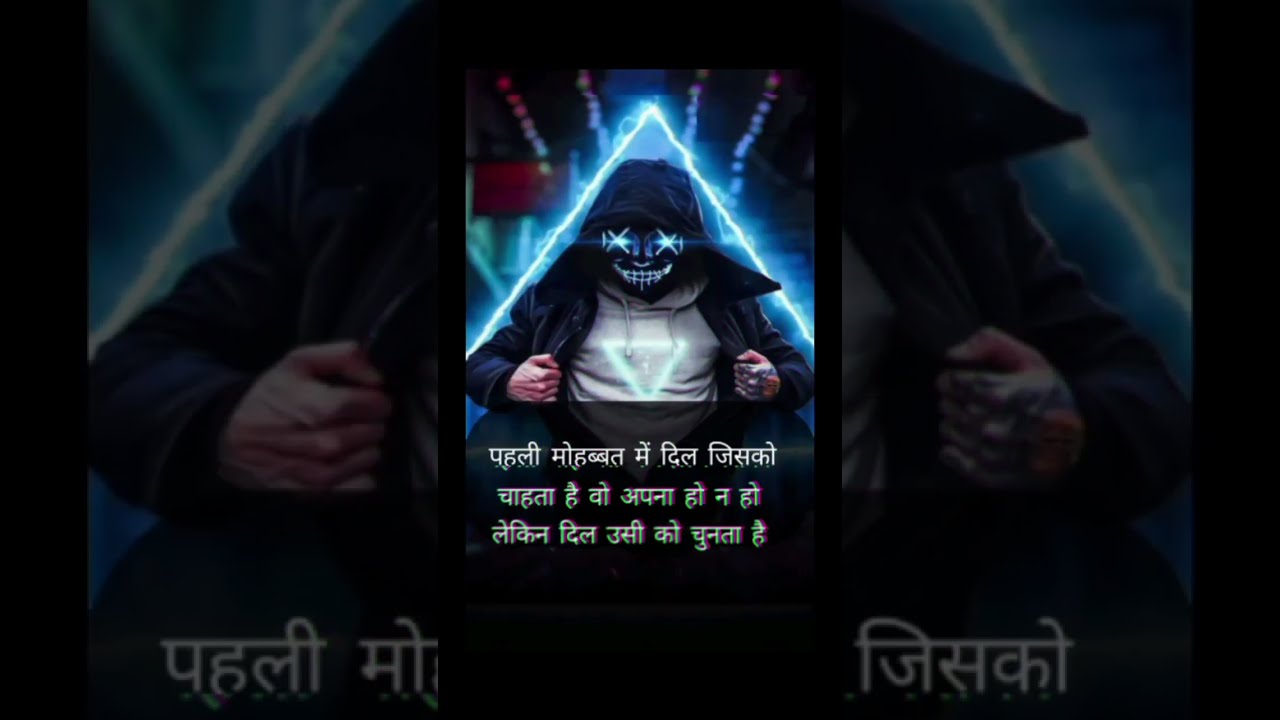The image depicts a vertical, comic-style illustration of a man wearing an open black hoodie, revealing a light gray or white sweatshirt underneath. His expression is monstrous, featuring a black mask or face with white stitches forming an X over each eye and a stitched, wide toothy grin. His eyes emit a glowing, whitish-green or blue light. He is clenching his fists and holding his coat open, showcasing an upside-down glowing blue triangle on his chest. Surrounding him is an electrically sparkling, right-side-up blue triangle emanating from above, forming a dynamic background element. Subtle, faded lines stick out from above his head. The scene is accented by a faintly visible, darkened, and zoomed-in version of the same image used as a backdrop. Below the figure, within a dark gray opaque box, is a three-lined text in white Arabic or Hindu script, featuring some chromatic aberration and progressively fading from the top down.